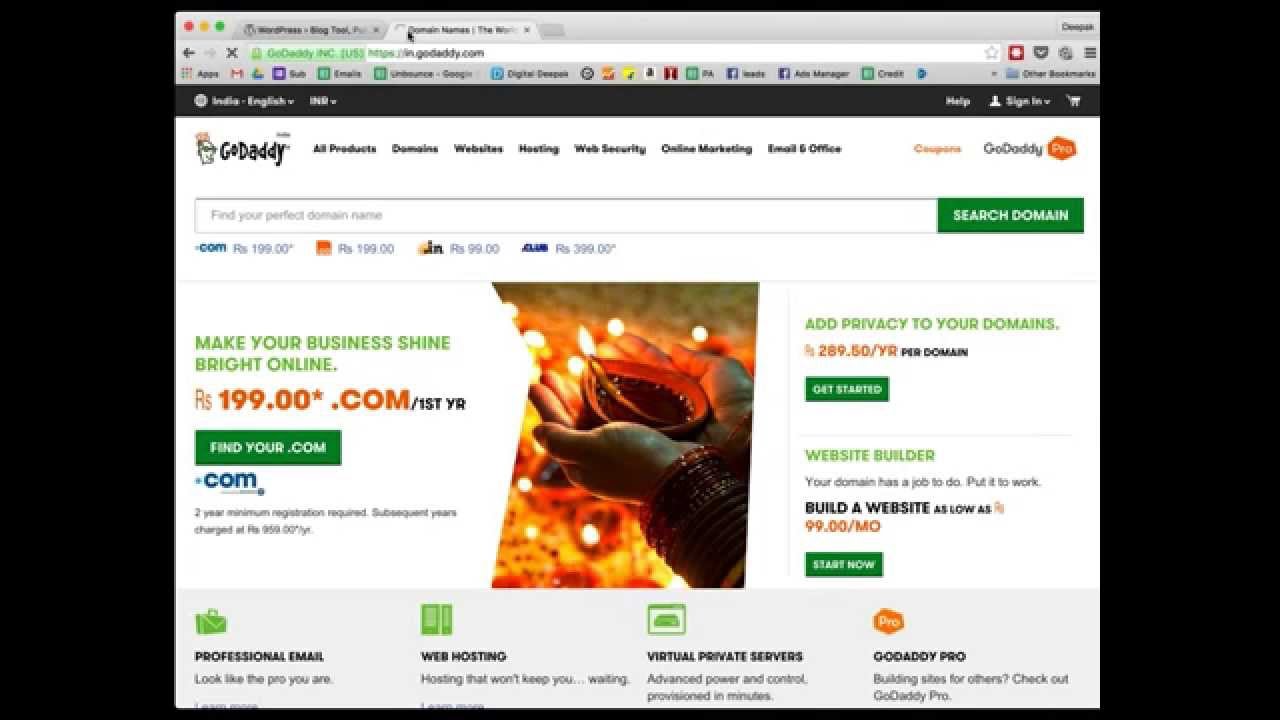**Detailed Description:**

The image is a screenshot displaying a webpage on a Mac browser. The browser has multiple tabs open, with the active tab being GoDaddy.com. The first tab, which seems to be related to WordPress, is not clearly visible. Below the tabs, there is a row of bookmarked icons.

At the top of the GoDaddy webpage, on a dark gray bar, there are options for language selection (likely English) and help. The page prominently features the GoDaddy logo, followed by a navigation menu with categories including All Products, Domains, Websites, Hosting, Web Security, Online Marketing, Email, and Office. Additionally, "GoDaddy Pro" is displayed within the logo on a white background.

Beneath the navigation menu, there is a large search field intended for domain searches, accompanied by a green search button with the text "Search Domain" in white.

Further down, the page advertises domain pricing, specifically mentioning ".com" domains for ₹199 for the first year, with currency appearing to be in rupees. The advertisement features an image of a person holding a candle, adorned with bracelets on their left arm, suggesting a Diwali-related theme.

The content includes various options like "findyour.com" and "greenbutton.com," but the details are blurred and compressed, making them difficult to discern. On the right side of the page, there is an offer to add domain privacy for ₹289.50 per year, with a call-to-action button "Get started."

Additional offers include website building services starting at ₹99 per month. At the bottom, four sections are highlighted: Professional Email, Web Hosting, Virtual Privacy, and GoDaddy Pro, each with corresponding logos.